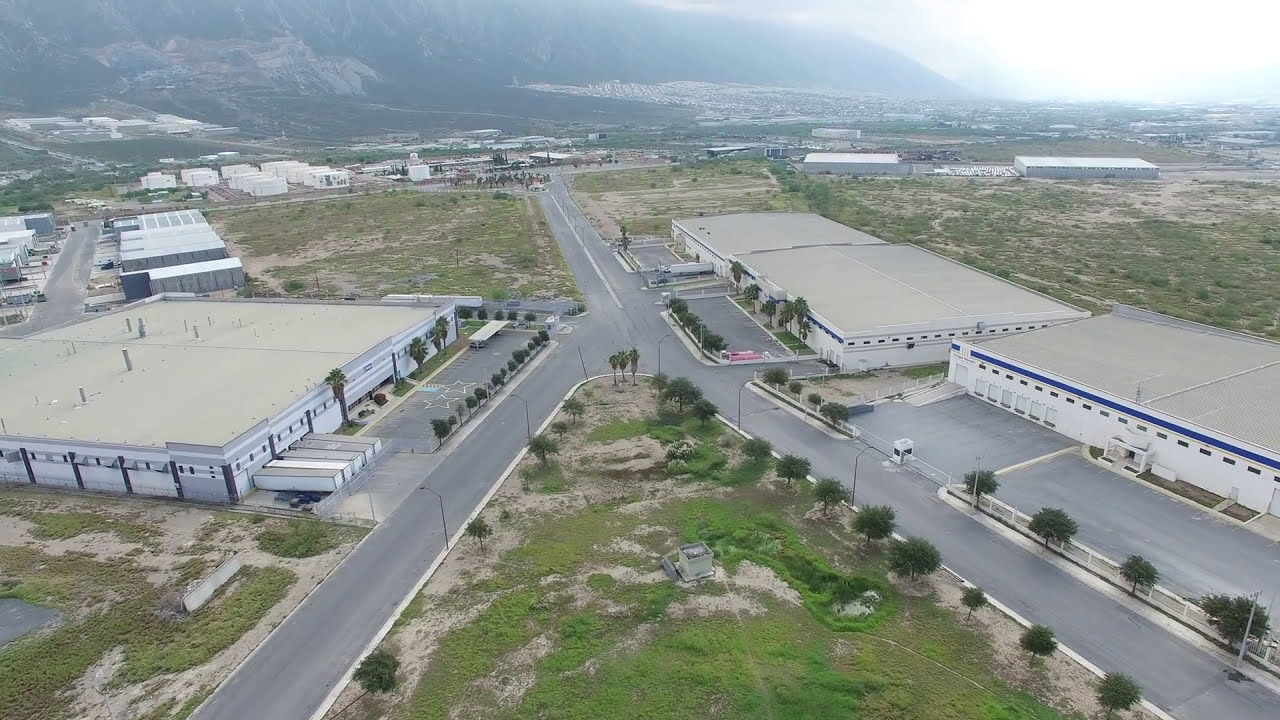This image captures a Y-shaped roadway junction from an overhead perspective, with the Y oriented upside down. On either side of the road, there are large, single-story, square white buildings that resemble warehouses or factories. The materials and colors suggest a semi-desert landscape, with light tan, dried-out grass and dirt surrounding the buildings and roadways. A triangular island of grass, trees, and dirt is prominent at the center of the junction. The scene includes scattered elements and uncentered placement, contributing to a sense of spaciousness.

In the background, a range of hills or mountains can be seen under a bright sky, with additional smaller buildings situated between the mountains and the junction. The planted trees along the roadway contrast with the otherwise dry, semi-desert environment. The photo, devoid of any visible text, conveys an outdoor setting in the middle of the day with colors like gray, white, green, tan, brown, yellow, red, and blue enhancing its vividness. The general impression is one of a sprawling, industrial-like complex within a semi-arid field, blending natural and manmade elements.